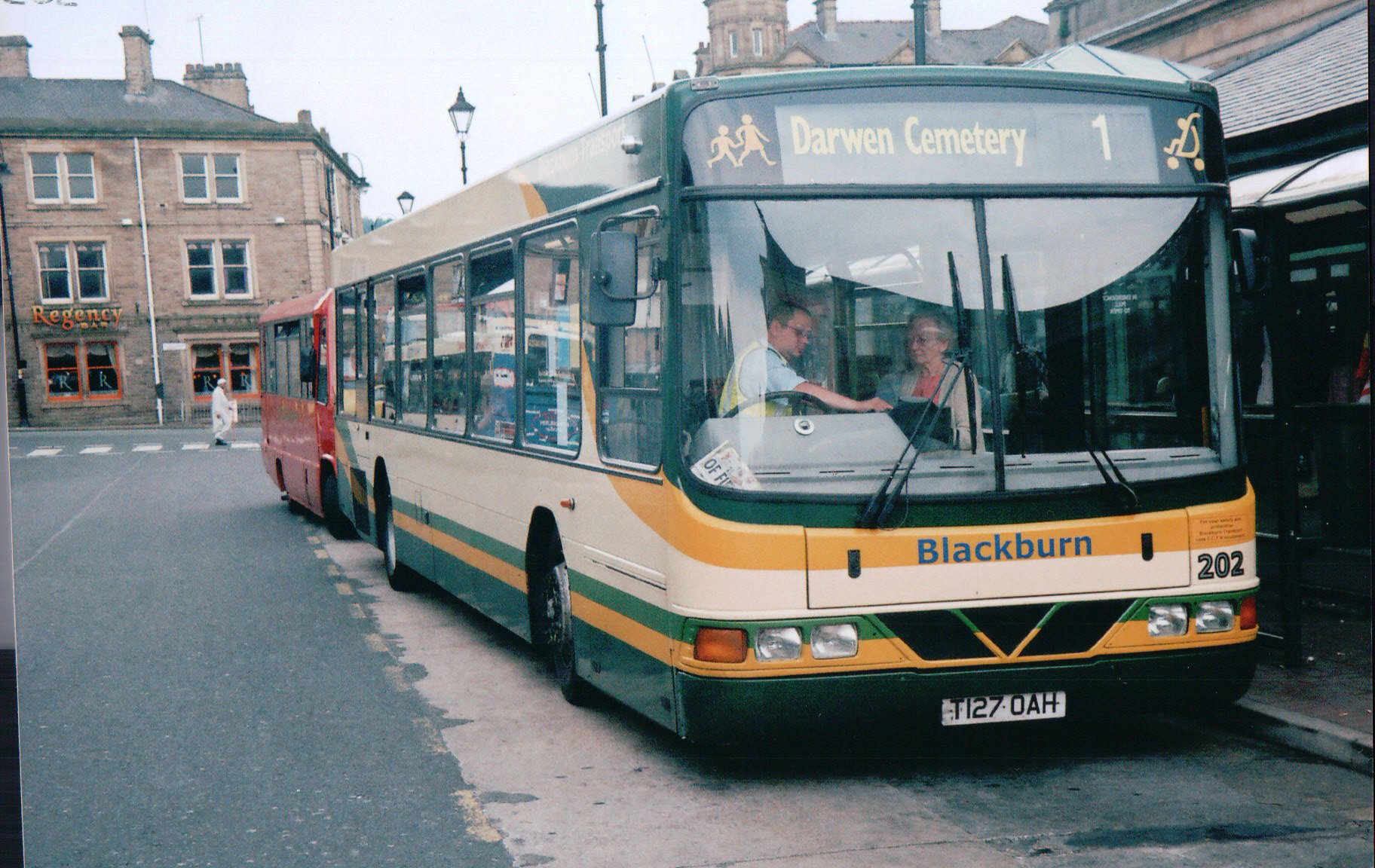The image captures a detailed urban scene with a vibrant focal point featuring a single-decker bus adorned in cream, yellow, and green colors. The bus prominently displays "Darwin Cemetery, number one" at the top left corner and "Blackburn" in blue text on the front, accompanied by the registration plate T1270AH. A driver, visible at the front, is engaged in conversation with a passenger standing inside the bus. Behind this bus, another single-decker bus in red can be seen. To the left of the red bus, a zebra crossing is traversed by a man in white clothing. The background features a three-story building with "Regency Bar" written in red and orange lettering, contributing to the atmospheric and realistic depiction of the urban setting.